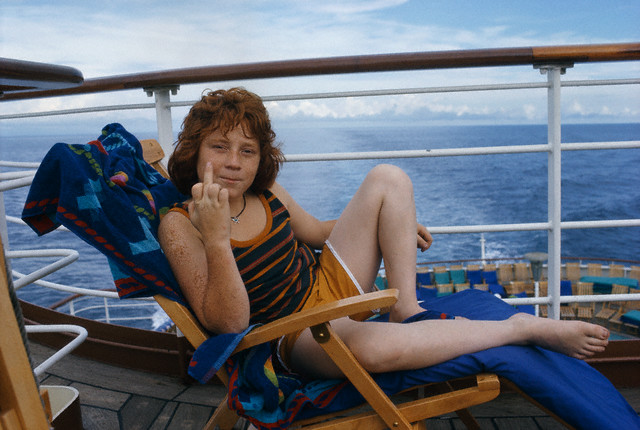The image captures a young person with long, curly red hair, which falls to their shoulders. They are lounging on a wooden chair on the deck of a boat or cruise ship. The individual is wearing orange shorts and a blue and orange striped tank top with an orange collar. They are seated on the chair with their left knee bent up, facing towards the right side of the picture, but their face is turned towards the camera, giving a bold gesture. The chair has a blue cushion and a blue towel is visible underneath them. In the background, you can see the boat's deck with its railing, along with the expansive ocean and distant clouds. There also appears to be a city skyline in the far distance.